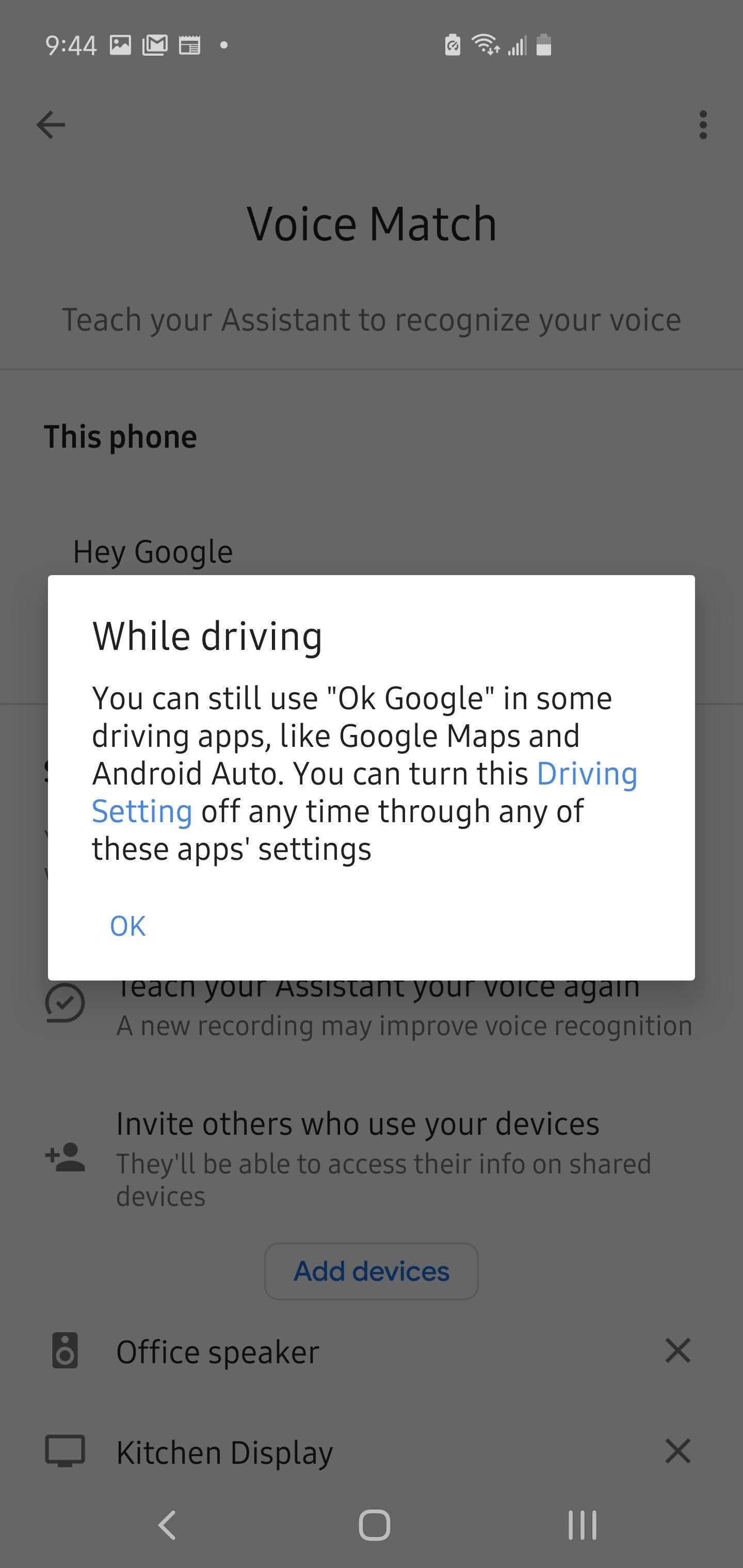This is a detailed screenshot of the Google Home setup screen. The background features a black semi-transparent overlay, indicating the presence of a pop-up dialog at the center. The pop-up is a white box with various informational sections. 

At the very top of the box, in bold black letters, it reads "While driving." Below this, in slightly smaller text, is a message explaining that you can still use "OK Google" within certain driving apps such as Google Maps and Android Auto. This can be controlled by adjusting the "driving setting," a phrase highlighted in blue. 

Further up in the pop-up, the section titled "Voice Match" is displayed in black letters. The caption below explains how to teach your Assistant to recognize your voice. To the left, there is a bold label, "This phone," followed by a description underneath that states, "Hey Google," indicating the voice activation command.

The pop-up overlays the central area of the background screen. Toward the bottom part of the background, bold text reads "Invite others who use your devices." Below this, it mentions, "They'll be able to access their info on shared devices." Centrally located at the bottom of the pop-up is a button with blue text that says "Add devices." The lower portion of the screen mentions specific shared devices, including "Office speaker" and "Kitchen display."